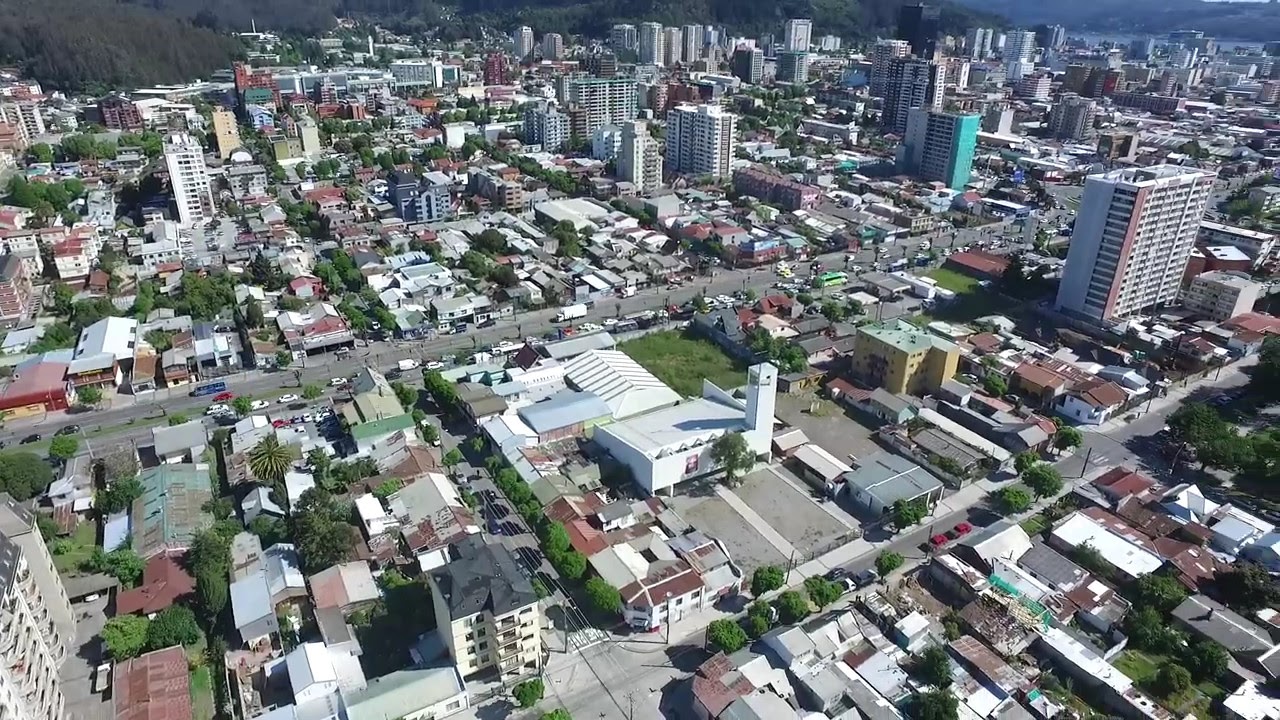This detailed aerial photograph showcases a modest cityscape, reminiscent of areas in Houston, Texas. The image is taken from a drone, providing a landscape-oriented view from above. The city features a mix of architectural styles, with numerous buildings ranging from 15 to 20 stories tall. High-rise apartments with white facades and scattered vegetation, including trees and bushes, make the scene quite green. The city’s layout includes a grid of intersecting streets with various colored rooftops—red, white, and blue—adding to the visual complexity.

In the bottom left corner, a neighborhood with single-story houses contrasts against the taller structures. The main street, equipped with streetlights and stoplights, runs through the city with four lanes, two in each direction. An apartment building about four stories tall is noticeable at the bottom of the photo, standing near the base of a mountain range with cliffs edging towards the city.

In the upper right corner, a body of water, possibly an ocean inlet or lake, is visible, adding a natural element to the urban landscape. Near this water body are a few high-rise buildings in a light gray finish. Centered in the image, an aqua-colored building stands out against its surroundings. The top left corner reveals a lush, forested area, completing this vibrant, realistic depiction of city life from an aerial perspective.